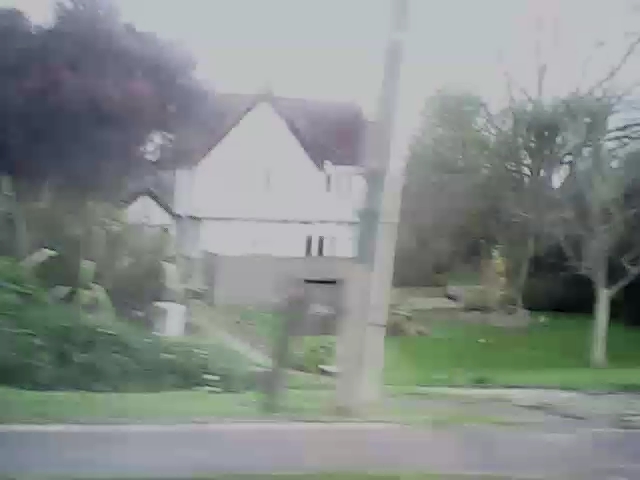The photograph is blurry, giving the impression that it might be AI-generated or a composite of different images. The background is light-colored with a smoky haze. In the middle of the scene is a white barn with a triangular, peaked front roof, contrasted by a darker rear roof. To the left of the barn is a dark deciduous tree. In front of the barn, there's a wall that appears to be part of an enclosed patio or first-floor wall. Surrounding the barn is green grass and several leafless trees. On the left side of the image, things get peculiar: there's a slight hill with gravestones that seem out of place, both in terms of proportion and the different shade of green grass. Dominating the foreground is a mysterious silver beam, leaning slightly to the right with segmented sections and a smaller beam extending to the left near the bottom, adding to the overall confusion of the scene.